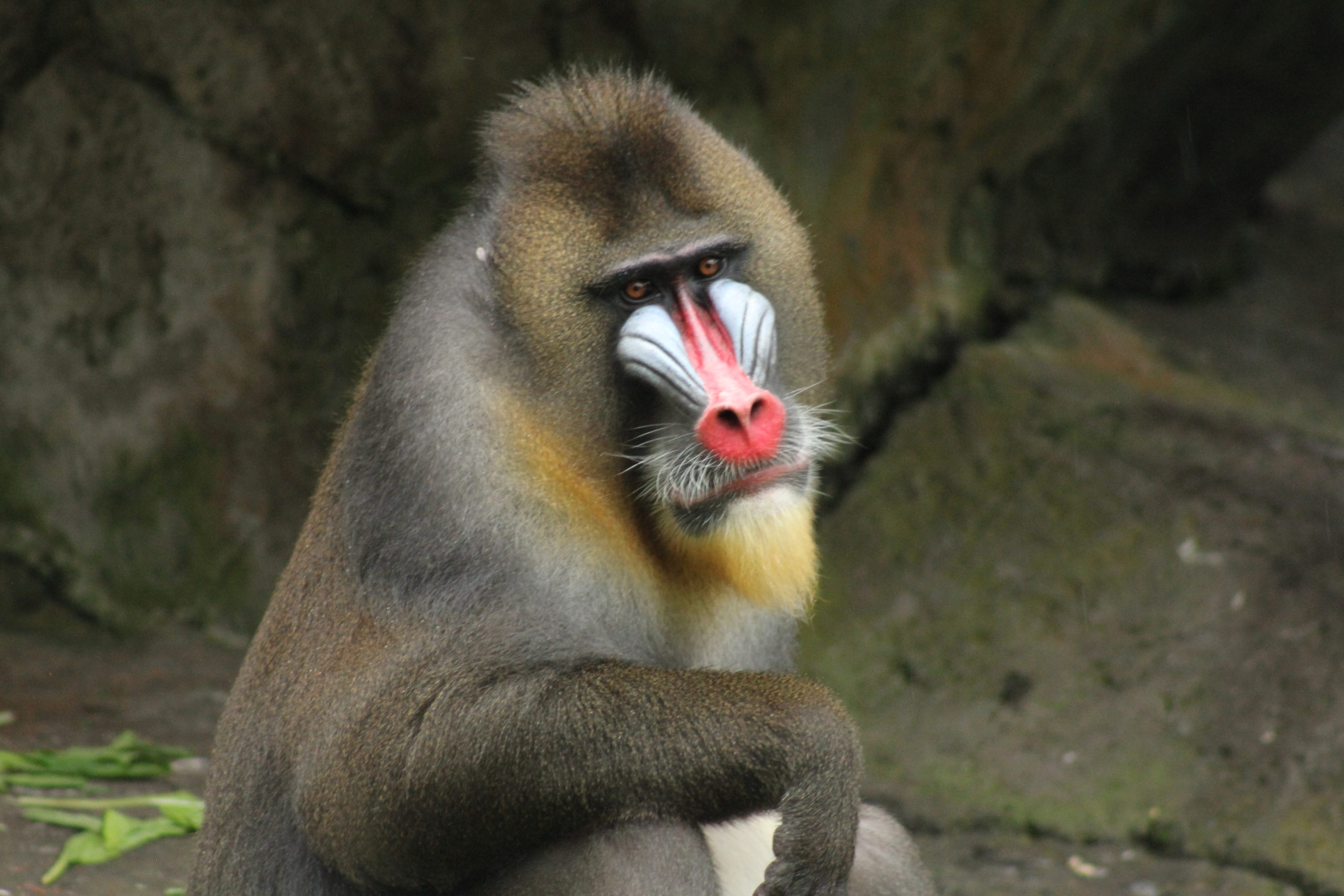A detailed close-up of a monkey, possibly an orangutan, is depicted in the image. The monkey features a distinctive reddish-pink nose with visible nostrils. Its cheeks are notable for their white hue, interspersed with small dashes. The monkey's eyes are a captivating reddish-brown, framed by white whiskers around its nose. Below its nose, the lips and a small white and orange beard are visible. The fur covering its body exhibits shades of brown and black. The monkey appears to be resting one paw on its knee and has its head slightly tilted. The background showcases a stone environment with a mix of brown and green tones, accompanied by some leaves in the bottom left corner.